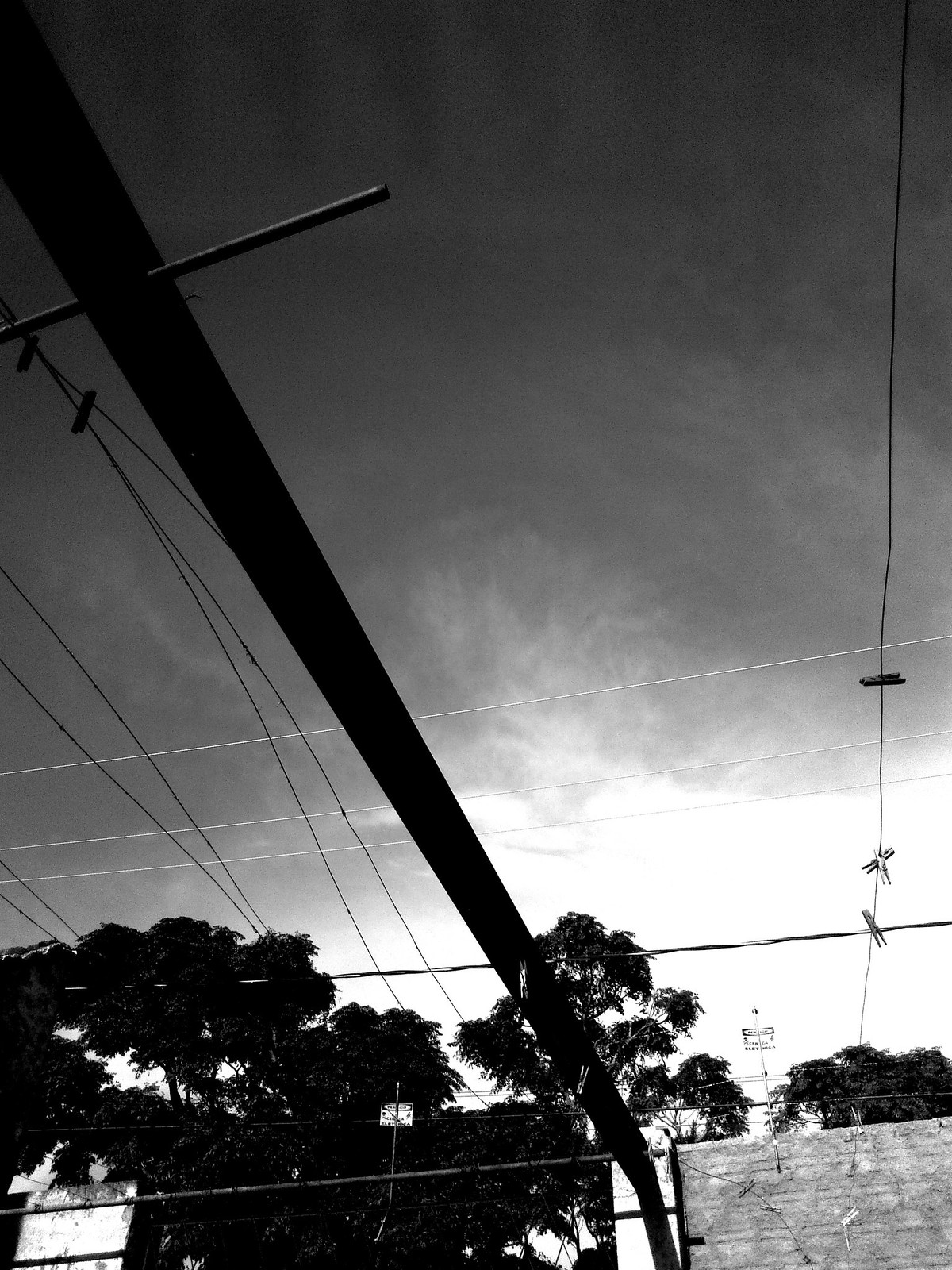This black and white photograph features a complex network of telephone wires extending both horizontally and vertically across the sky, which is filled with dark gray clouds. The image appears to be taken from a low angle, as if the photographer was lying on their back, causing the sky to dominate the upper two-thirds of the composition. In the foreground, there is a cluster of tall trees, their tops silhouetted against the sky, and a brick building partially visible in the bottom right corner. A sign is attached to one of the wires, adding to the intricate interplay of lines. The bottom third of the image also includes a tall wall, adding a sense of boundary. Additionally, a clothesline with clothespins, but no clothes, stretches across part of the scene. The photograph has an abstract quality, emphasizing the stark, intersecting lines of the poles, wires, and trees, creating an almost industrial atmosphere that suggests it could be near a train station or power area.